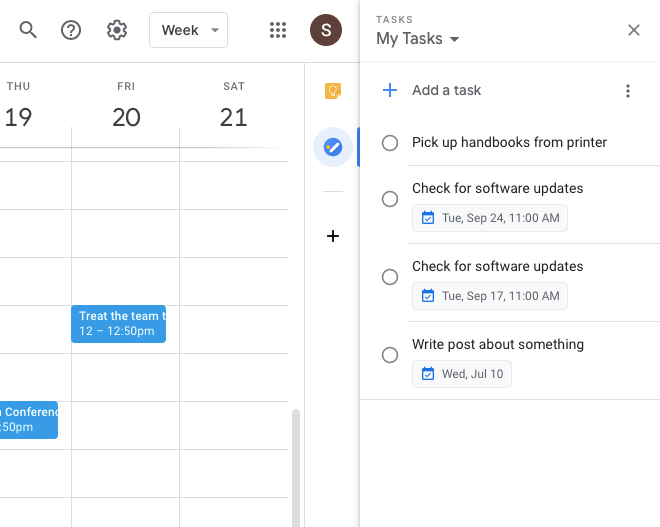This image appears to depict a task management interface, possibly from a web application or a mobile app. At the top left corner, there are three icons: a magnifying glass (likely for search), a question mark inside a circle (for help or information), and a gear (for settings). To their immediate right, there is a dropdown labeled "week" with a down arrow next to it. Further right, there's a brown circle with a white letter "S" inside, presumably a user profile icon.  

To the right of the profile icon, a prominent section labeled "Task, My Task" features another dropdown menu indicated by a down arrow, and an "X" for closing the section. Below this section is an input area labeled "Add a Task," accompanied by a blue plus symbol. Four tasks are listed beneath this: 

1. "Pick up handbooks from printer."
2. "Check for software updates," scheduled for Tuesday, September 24th at 11 am.
3. A duplicate task, "Check for software updates," scheduled for Tuesday, September 17th at 11 am.
4. "Write about something," set for Wednesday, July 10th.

To the left of these tasks is a calendar-like section displaying dates: Thursday the 19th, Friday the 20th, and Saturday the 21st. Overlaying this calendar area, there is a grid with both horizontal and vertical lines, likely representing a Gantt chart or a schedule grid.